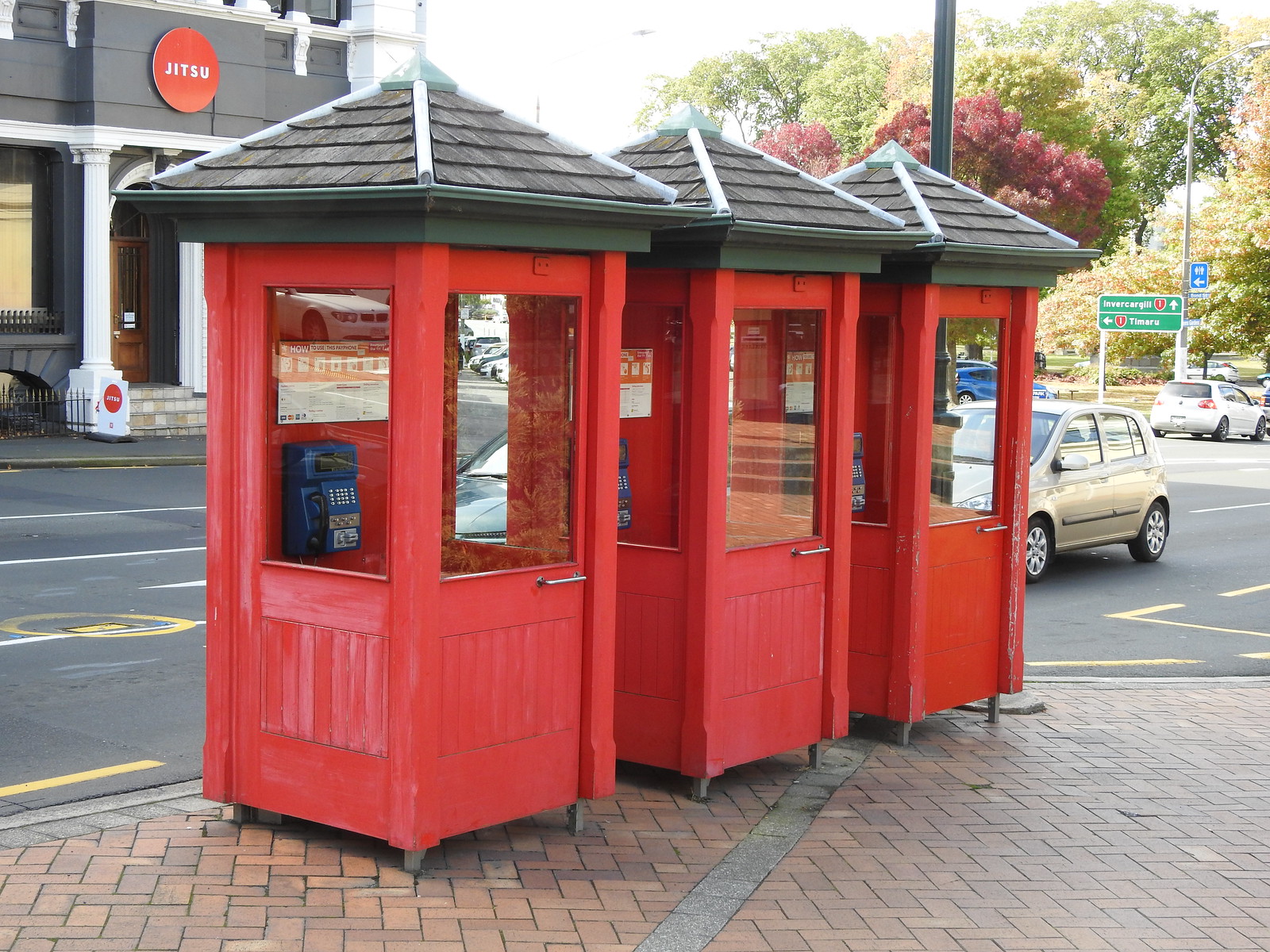The image captures a vibrant street scene set in what appears to be a foreign country, possibly China. Dominating the foreground are three striking red wooden telephone booths, styled to resemble traditional pagodas, complete with shingled, pagoda-like grey roofs. Each booth features four glass windows per side, providing a clear view of the large payphones mounted inside, which come with detailed usage instructions.

These telephone booths are neatly aligned along the edge of a sunny sidewalk, indicating it's autumn as evidenced by the trees with turning leaves, particularly a maple tree showcasing vivid red foliage. A gold car is seen approaching from the right side of the photo, about to pass behind the booths, emphasizing the busy street setting. Further detailing the backdrop, a modern, grey building with a large sign that reads "Jujitsu" is visible across the street, contributing to the scene's mix of traditional and contemporary elements. The road in front appears well-paved, and cars intermittently drive back and forth. A stop sign with partially readable text, possibly "trim," stands in the distance, adding to the urban landscape's layered details.